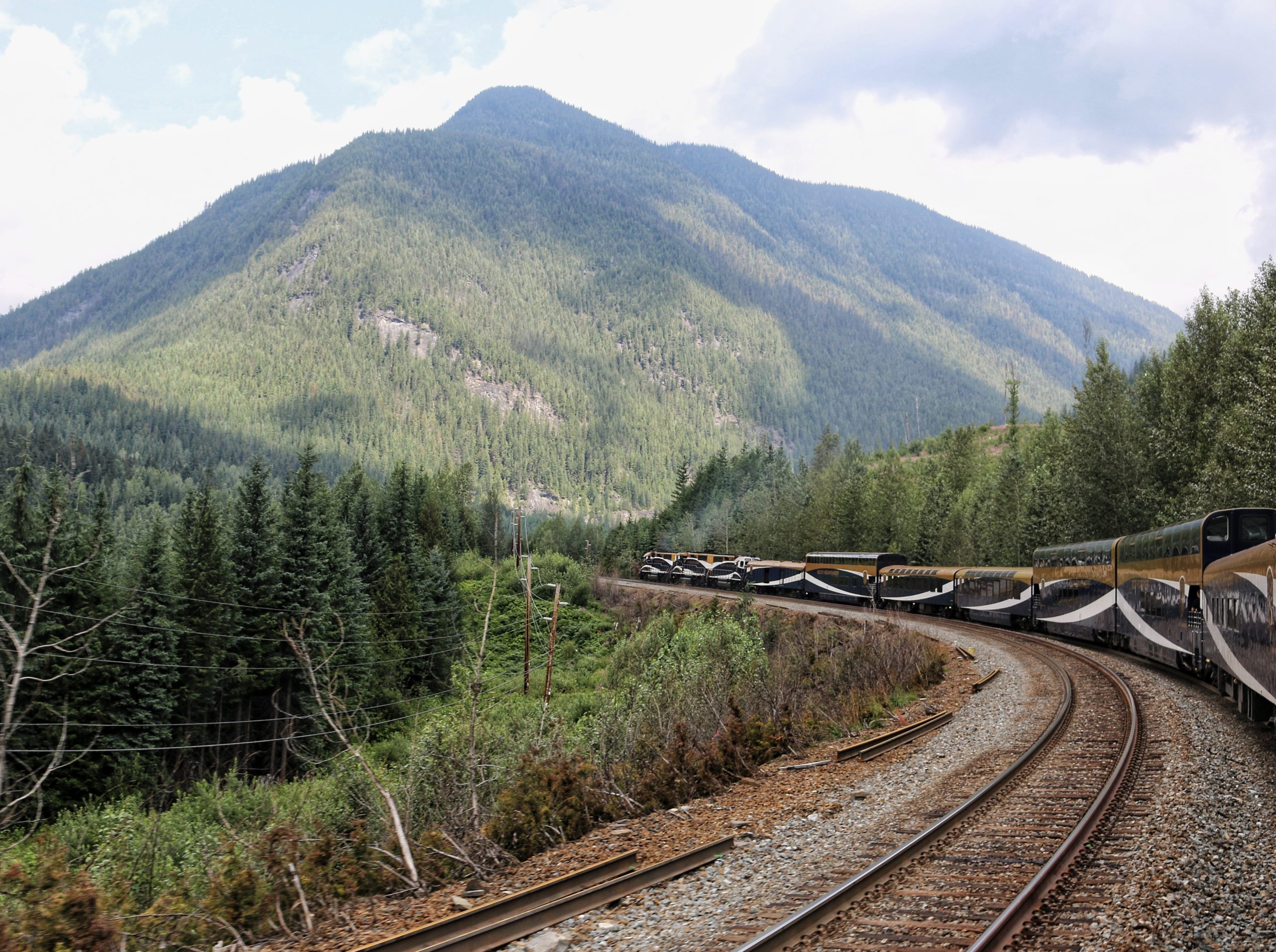This photograph features a scenic landscape where railroad tracks stretch prominently in the foreground, curving to the left and leading the viewer's eye towards a distant, majestic, forested mountain. The mountain, dotted with patches of sunlight and shadow created by fluffy white clouds, stands tall under a partly blue sky. The train tracks on the right side are lined with steel rails and a series of black, white, and gold train cars with viewing boxes, producing steam as they head towards the viewer. To the left of the tracks, a series of electrical power lines and poles run parallel, flanked by lush trees and smaller foliage, further contributing to the picturesque setting. The photograph captures the tranquility of the daytime scene, with the sunlight illuminating the dense forest on the mountain, interspersed with occasional rocky outcrops peeking through the verdant greenery.